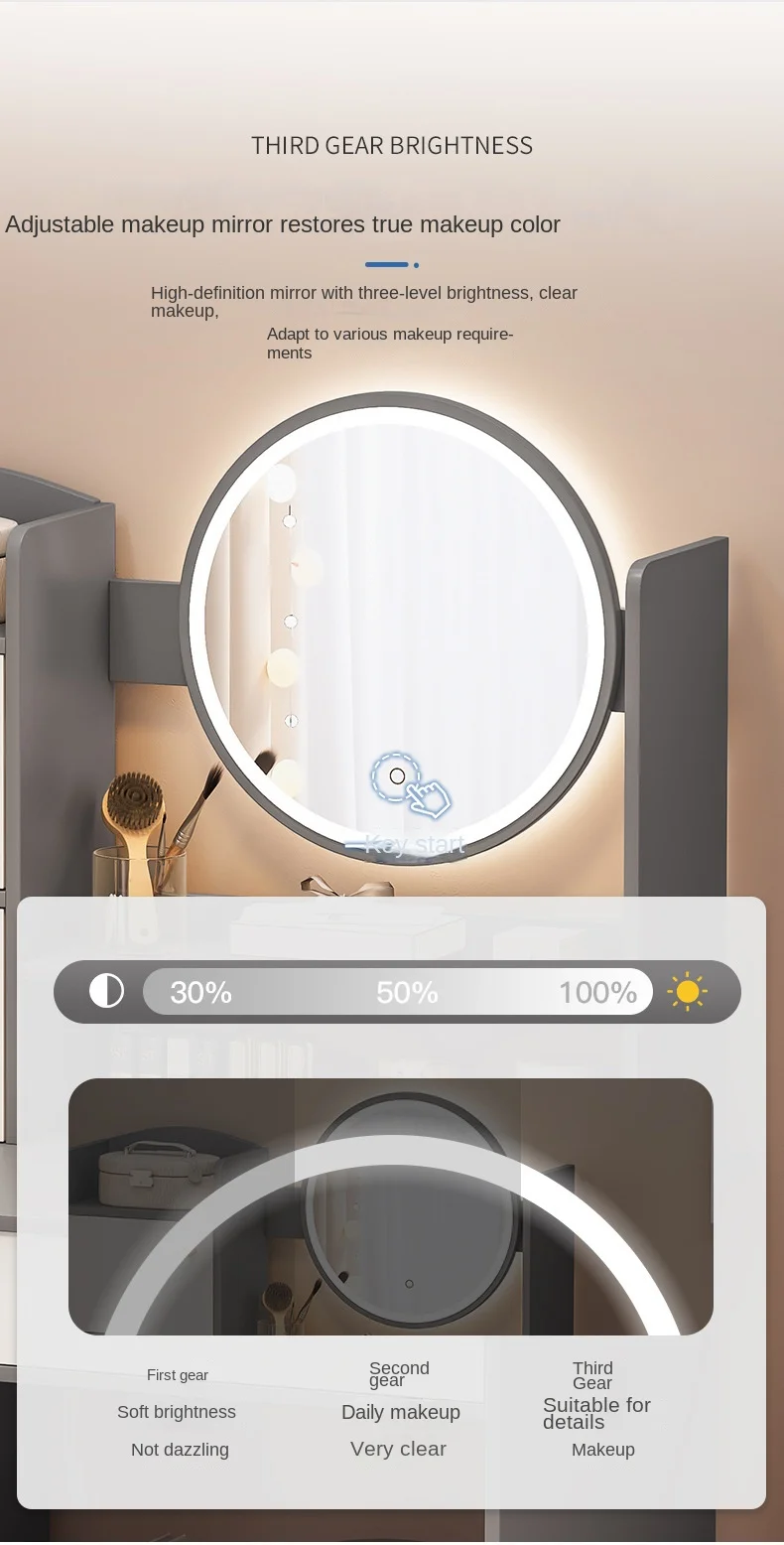This is an image of a product advertisement showcasing an adjustable makeup mirror designed to restore true makeup color. The mirror features high-definition clarity with three adjustable brightness levels to cater to various makeup needs. 

The circular mirror is equipped with integrated lighting in the center, enhancing visibility for precise makeup application. At the bottom of the mirror, there is a touch-sensitive button, depicted by a hand gesture symbol, allowing users to control the light settings.

Additionally, the advertisement details the adjustable brightness levels with a graphical representation. A bar at the bottom left displays 30% brightness, the middle section shows 50% brightness, and the right side indicates 100% brightness. Another visual bar represents the light's intensity range, illustrating a progression from a grey color to a silver tone, and finally to a clear, bright light. Corresponding labels at the bottom categorize the brightness settings as "First Gear," "Second Gear," and "Third Gear."